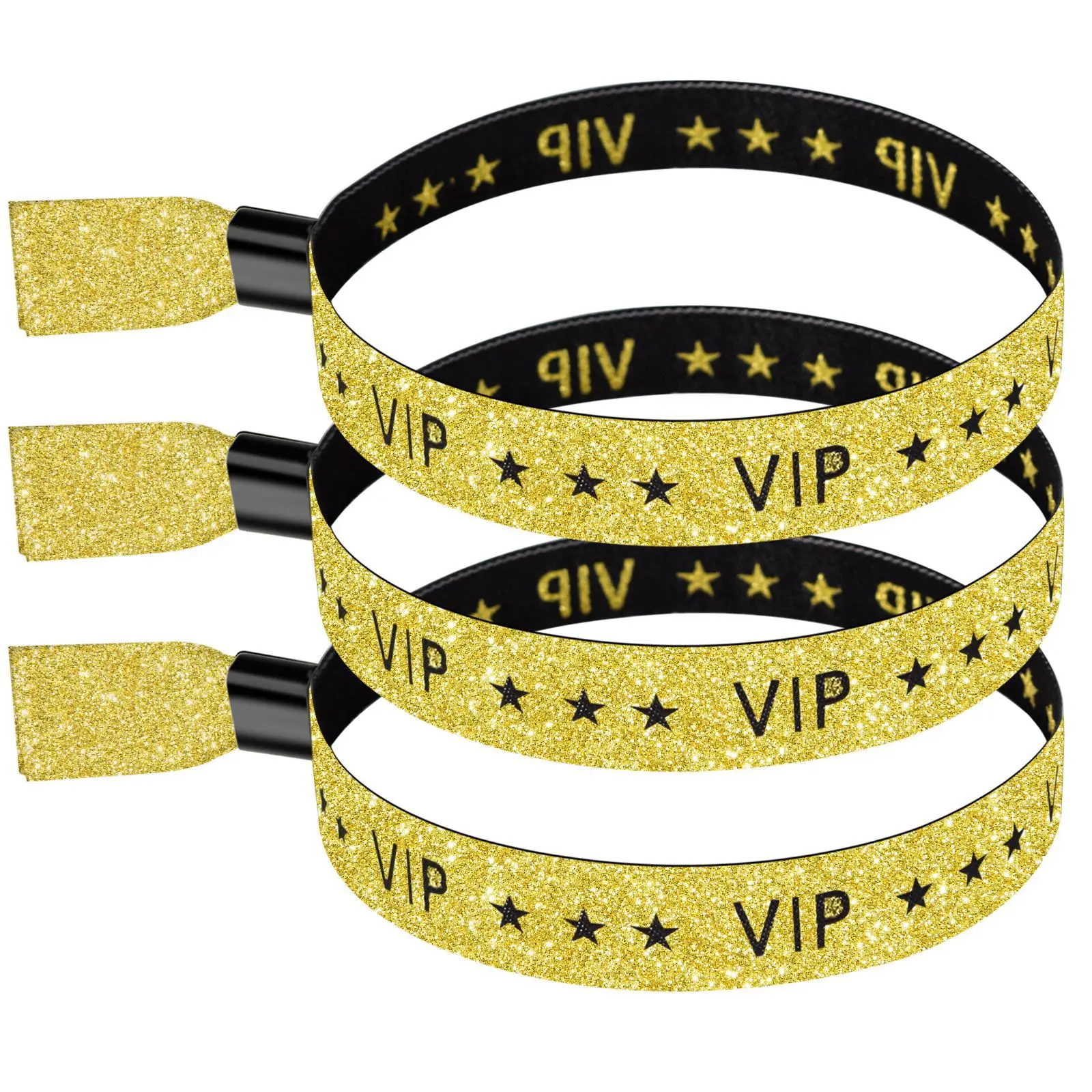The image showcases a set of three intricately designed bands, which could be utilized as either headbands or wristbands. Each band prominently displays the word "VIP" in bold black letters against a shimmering gold background, embellished with three stars, signifying exclusivity. On the inside, the word "VIP" is also inscribed, but in luxurious gold lettering set against a sleek black background, maintaining the motif of prestige. Near the edges of each band, there is a black clip mechanism designed for adjustable sizing, adding a functional and stylish element to the accessory. The bands appear to be part of a promotional campaign, likely aiming to convey a sense of luxury and exclusivity. The image itself is strikingly detailed and rendered in 3D, giving it a lifelike quality that suggests it may be a high-quality photograph or a computer-generated graphic. The intricate detailing and the vivid contrast between the gold and black elements make this image especially eye-catching.